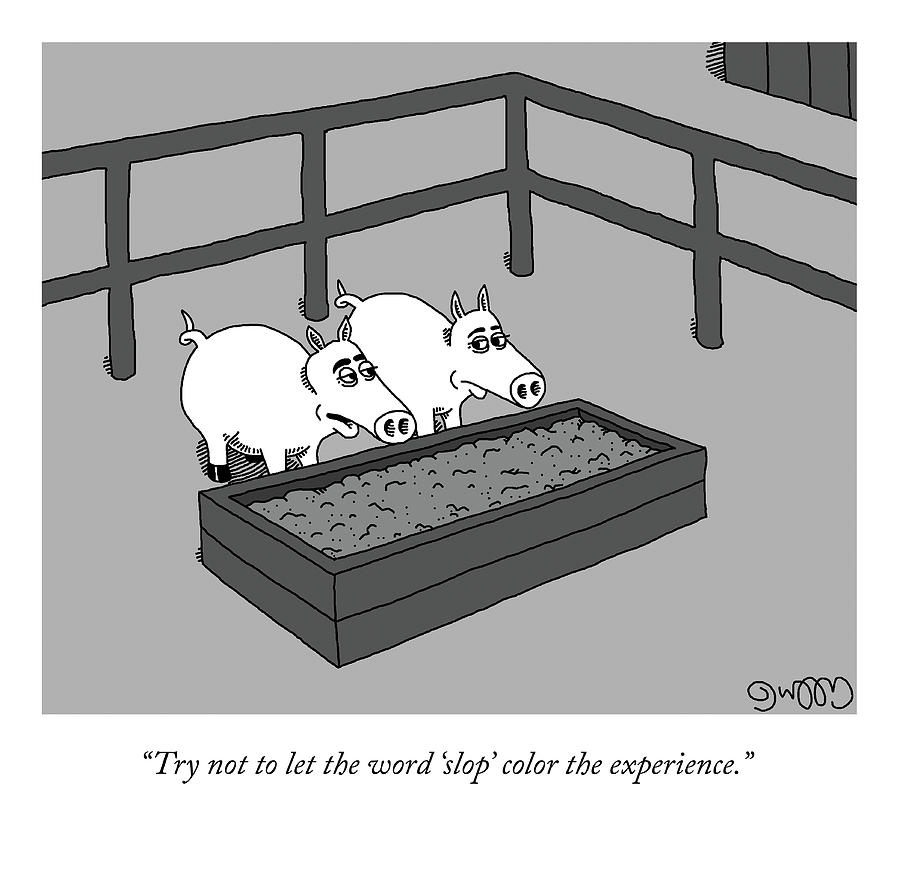This black-and-white cartoon features two anthropomorphic pigs with exaggerated human-like facial characteristics, including large eyes and eyebrows that convey expression. They are situated in a fenced pen with a dark gray railing, standing before a rectangular trough filled with a mush-like substance, likely referred to as "slop" in the context. The background includes the partial view of a wood-slat building in the upper right. Below the image on a white background is a caption in black text that reads, "Try not to let the word slop color the experience." A signature, potentially reading "W00D," is located at the bottom right of the image.